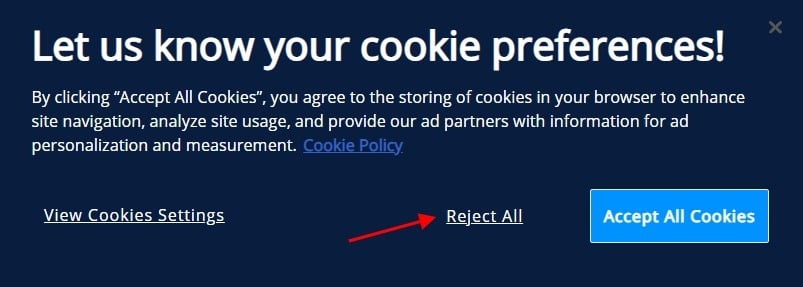The image is a pop-up for cookie preferences. It has a navy blue background and spans approximately three times as wide as it is tall. The text on the pop-up is in white, standing out clearly against the dark background. 

The header reads "Let us know your cookie preferences," followed by a paragraph explaining: "By clicking accept all cookies, you agree to the storing of cookies in your browser to enhance site navigation, analyze site usage, and provide our ad partners with information for ad personalization and measurements." 

In the center of the pop-up, there is a blue link labeled "cookie policy" for users to get more information. 

At the lower portion of the pop-up, three options are presented from left to right: 
1. "View cookie settings" in plain white text, without a button.
2. "Reject all," also in plain white text, but with a noticeable red arrow just to its left. The arrow points slightly upwards to the right toward this option.
3. "Accept all cookies," which is prominently displayed within a bright light blue button located at the lower right corner. 

A gray 'X' in the upper right corner allows users to close the pop-up.